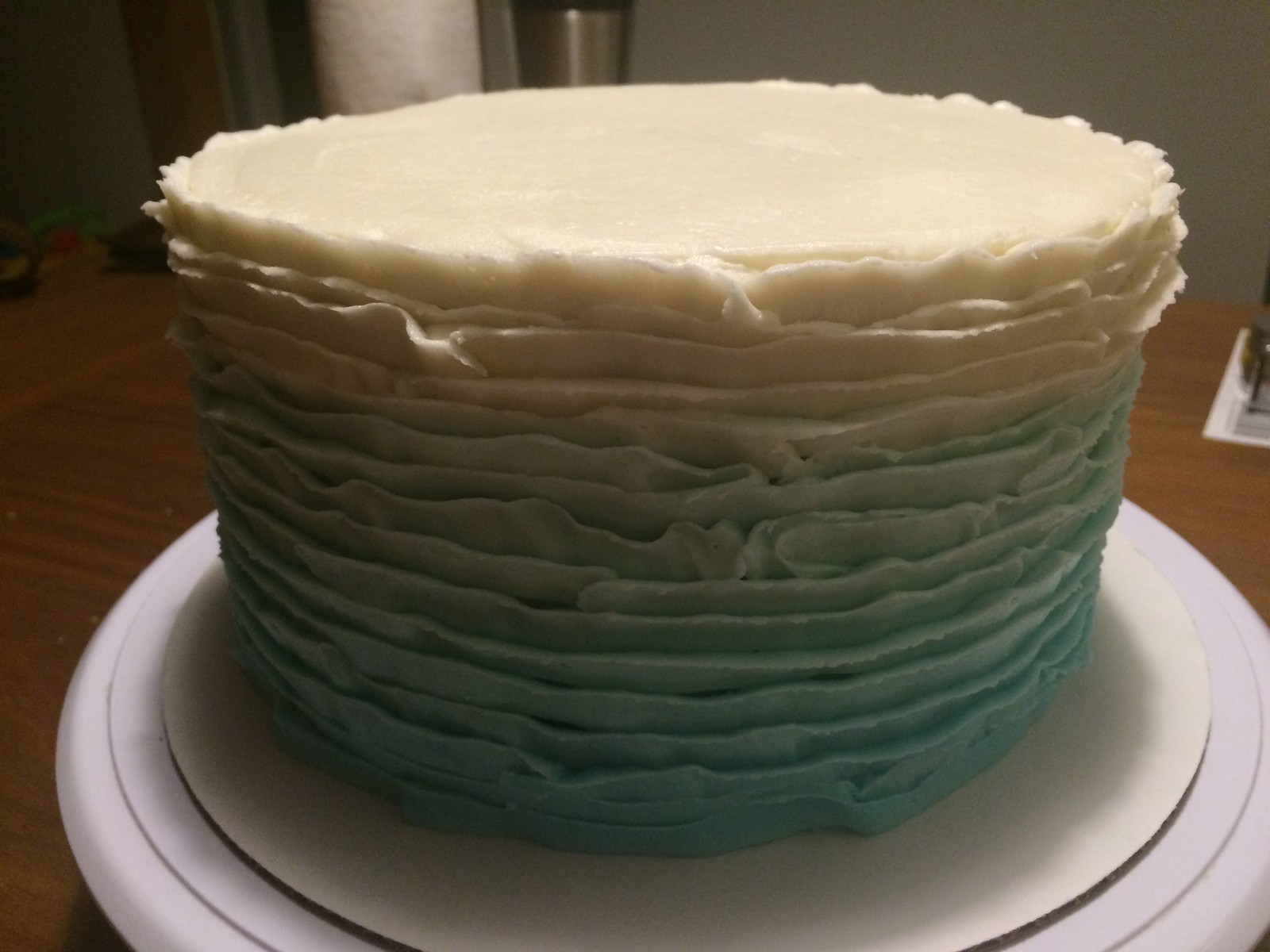The image depicts a close-up of a small, round cake, artfully frosted with a gradient from white at its smooth top to light green and finally to blue at its base. The frosting, likely buttercream, is skillfully applied in thin, layered ribbons that wrap around the circumference, creating a delicate textured pattern. The cake rests on a white plastic cake turntable, designed for easy rotation during decorating, which is in turn placed on a brown wooden table. A typical cardboard cake plate is seen underneath the cake, with its white top peeking out. The background features a partially visible silver cup and a white wall, hinting at a simple, unstaged setting. Lighting from above illuminates the cake, highlighting its intricate frosting details.